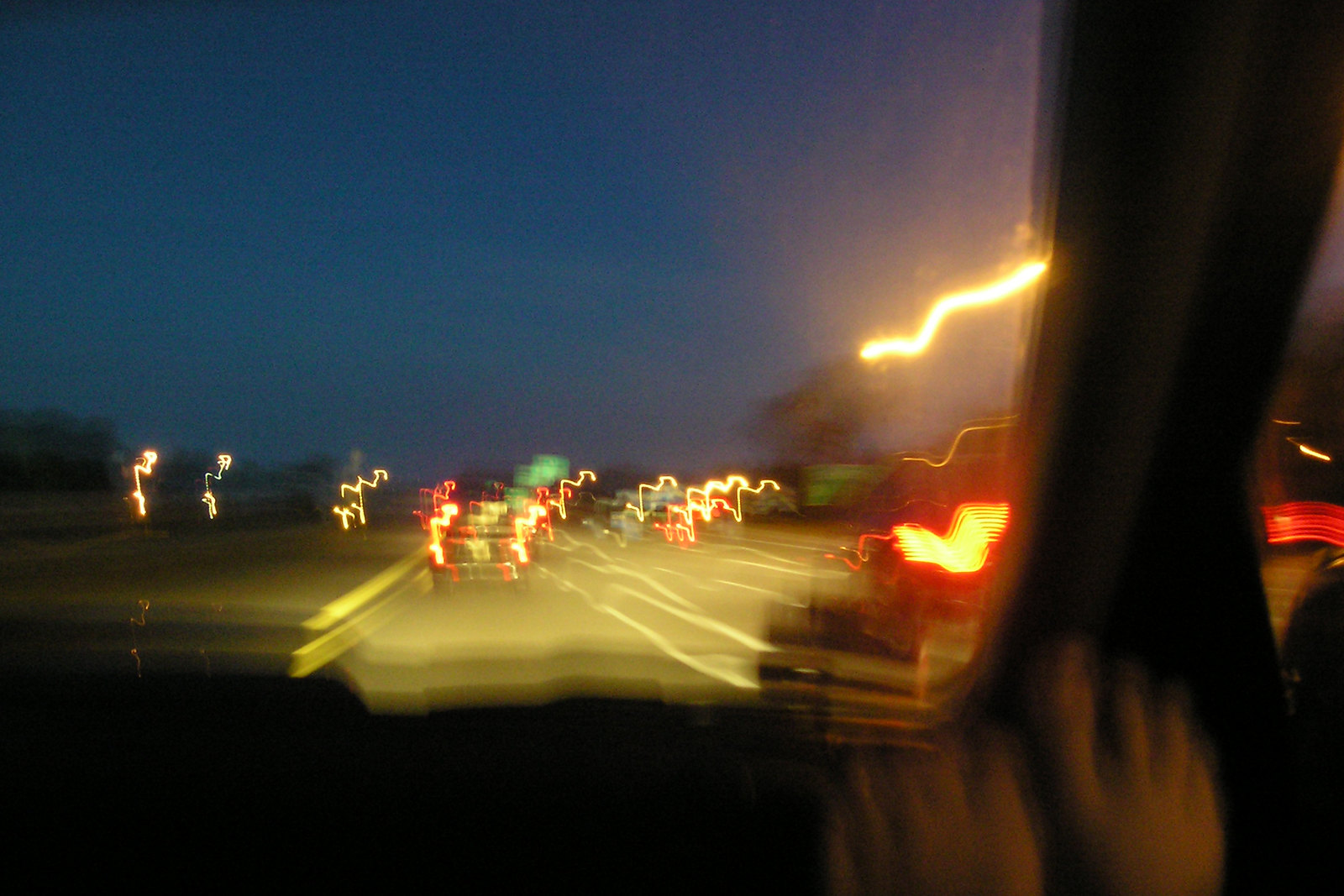The photograph captures a nighttime scene from inside a moving car, looking through the windshield onto a bustling highway illuminated by streetlights. The digitally enhanced image features dramatic zigzag, lightning-shaped light trails emanating from each light source, including the streetlights on the left side and the numerous taillights of the cars ahead. These striking light trails span from the bottom left to the top right of the frame, creating a surreal visual effect that emphasizes the motion. The shot is taken from the passenger's perspective, showing a semi-blurred view of bare feet propped up on the dashboard, with the toes slightly cut off due to the motion blur. The car's interior, including parts of the dashboard and the frame between the windshield and the passenger door, is visible, providing context to the chaotic outside scene. The blurred outline of another car and highway signs in the distance further add to the image's dynamic composition.